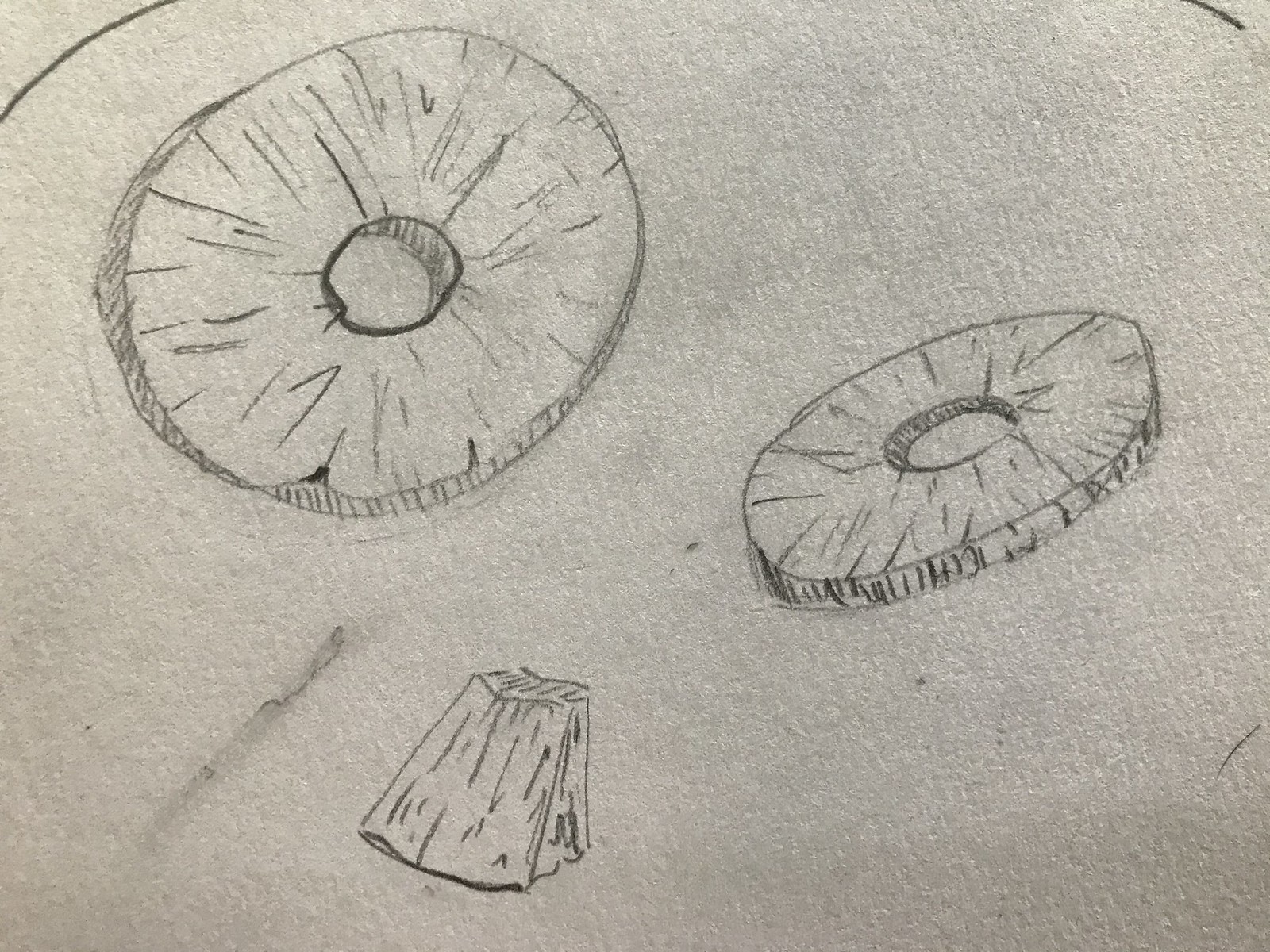This photograph captures a series of pencil illustrations rendered on a textured, white surface. The drawings exhibit a high level of detail and feature shapes that could be interpreted as either pineapple slices or wooden discs. The top-left illustration displays a 3D-rendered wheel-shaped object with intricate lines of detail, making the circular form and the cylindrical depth visible, giving it a thick, disc-like appearance. Below, another similar disc is depicted at a different angle, highlighting more of its side profile. At the bottom left, a smaller shape resembling a 3D trapezoid adds variety to the composition. The pencil work is meticulous, although the surface shows some smudges and dark spots, contrasting against the predominantly white background.